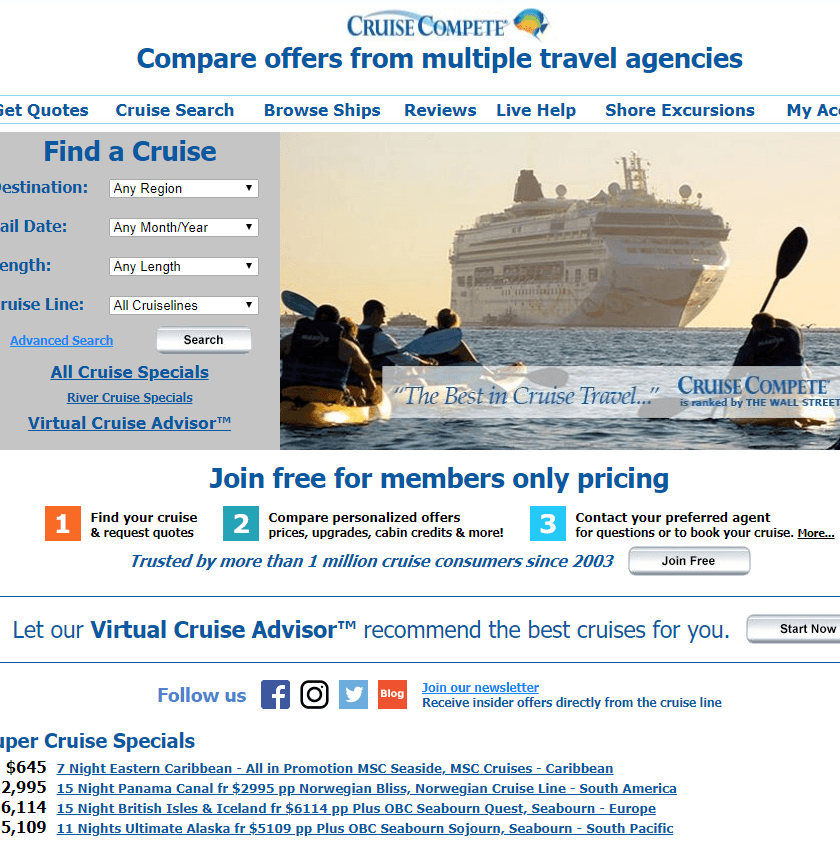A cropped screenshot from the Cruise Compete website, a platform for comparing cruise packages. The image features a dated 2000s-style design with grey, blue, and white color schemes. At the top, a search section allows users to look for cruises by destination, sail date, length, and cruise line. To the right of this search box, there's an image of a large ferry sailing on the sea. Beneath the search area, advertisements promote pricing deals, including a banner that says "Join Free for Members Only Pricing." Icons at the bottom link to social media pages on Facebook, Instagram, and Twitter (also known as X), along with hyperlinks to subscribe to the newsletter. The very bottom of the page includes additional links and prices for special cruise offers.